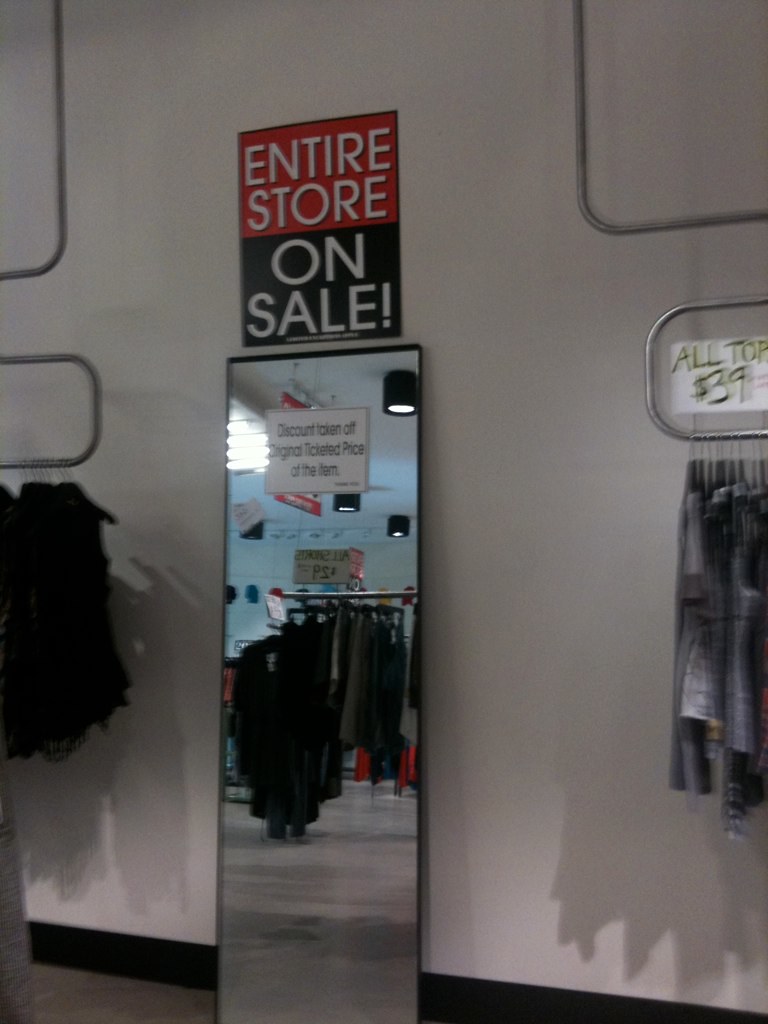This photograph captures the interior of a retail store amidst a sale event. Dominating the upper portion of the image is a bold red and black sign that reads, "Entire Store on Sale." Beneath the sign, a four-panel mirror is mounted against the wall, with a white paper note affixed, stating, "Discount taken off original ticketed price of the item." To the right of the mirror is a clothing rack showcasing a variety of tops, each priced at $39. Among these garments are short-sleeved denim tops. Adjacent to these are several black, sleeveless tops that resemble vests. The store’s floor is composed of plain concrete, while the white walls are accentuated by a black baseboard trim running along their bottom edges.